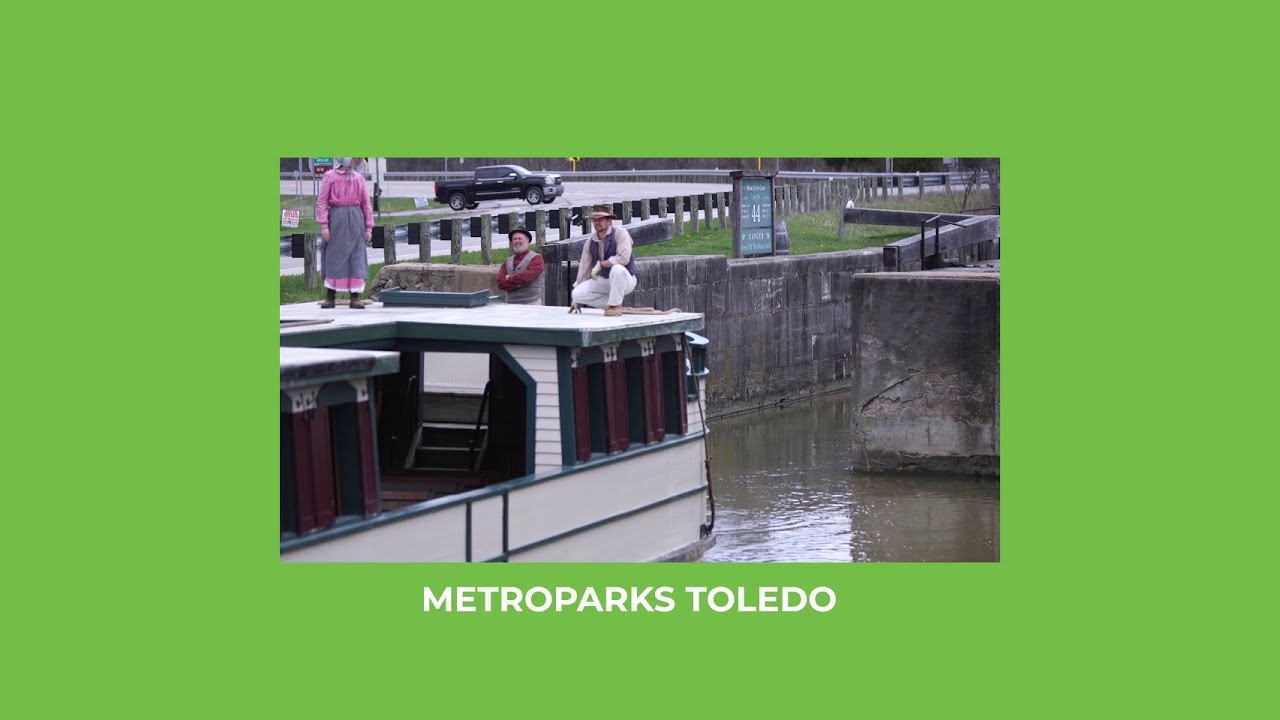This vintage-style photograph, framed in a thick green mat with the inscription "Metro Parks Toledo" at the bottom, showcases a riverboat on a waterway bordered by tall gray cement walls. On top of the boat, which features white sides, red window shutters, and a white roof, stand three individuals: a woman dressed in a pink dress with a gray apron, and two men wearing vests—one in a gray vest over a white shirt and pants, and the other in a gray vest with a burgundy shirt. The woman and one man are positioned on the upper deck, while the second man stands on a slightly lower level. In the background, a black four-door pickup truck is parked in a lot, backed into a spot separated by a metallic guardrail. A numbered sign "44" is visible on a stone wall that encloses the waterway.